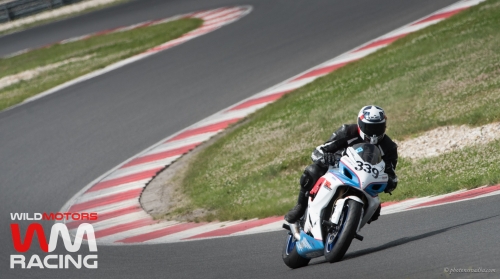The image depicts a motorbike racer navigating a winding, S-shaped track with red and white striped edges flanked by grassy areas on the interior curves. The asphalt course is predominantly black or gray. The rider is on a white motorcycle adorned with blue accents and the number 339 in black on the front. He is dressed in black gear, including a jacket, gloves, knee pads, and boots. His helmet is white with a distinctive blue circle and a large white star in the center of the top. The visor is down. In the bottom left corner, there is an advertisement for Wild Motors, featuring a logo that cleverly combines the letters W and M in red and white. The text reads "WILD Motors," with 'Wild' in white and 'Motors' in red, followed by "RACING" in all caps, white font.